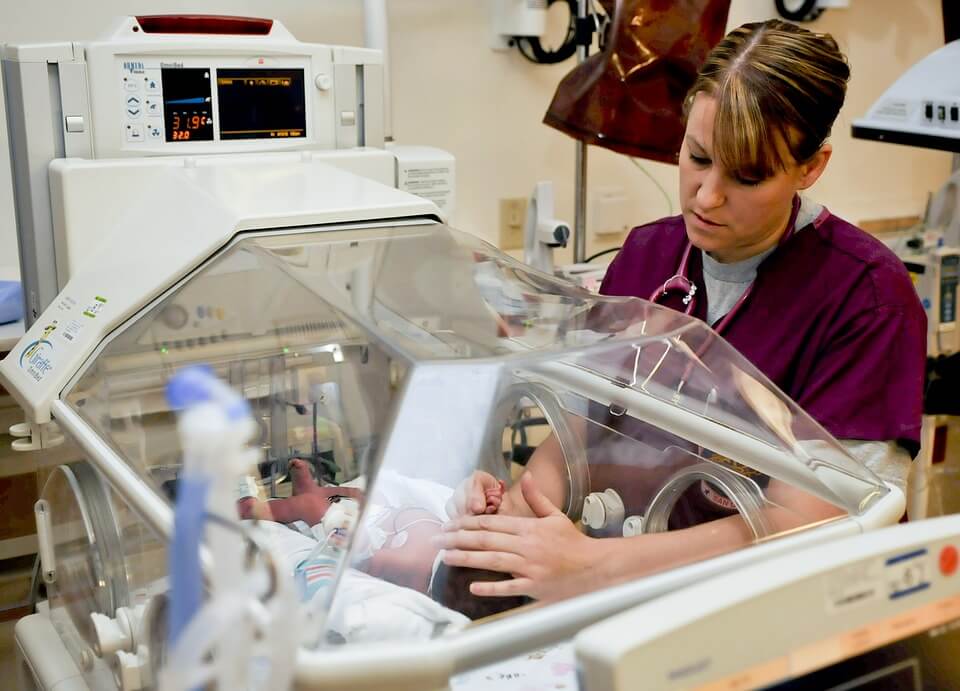This detailed photo captures a somber scene within a hospital room, likely in a neonatal or pediatric intensive care unit (NICU). The central focus is an incubator with a transparent case housing a frail infant, who appears to be born prematurely and in need of close medical attention. The baby rests inside the incubator, facing the camera with its tiny feet towards various medical monitors in the background. Positioned beside the incubator is a middle-aged nurse or doctor, diligently tending to the infant. She wears wine-colored scrubs over a gray undershirt and has a purple stethoscope draped around her neck. Her light brown and black hair frames her face as both of her hands reach through the incubator's openings to care for the baby. Behind her, a white device with a digital screen and several other essential machines emphasize the critical care environment. Her compassionate demeanor and methodical care exude a sense of dedication in this life-sustaining setting.